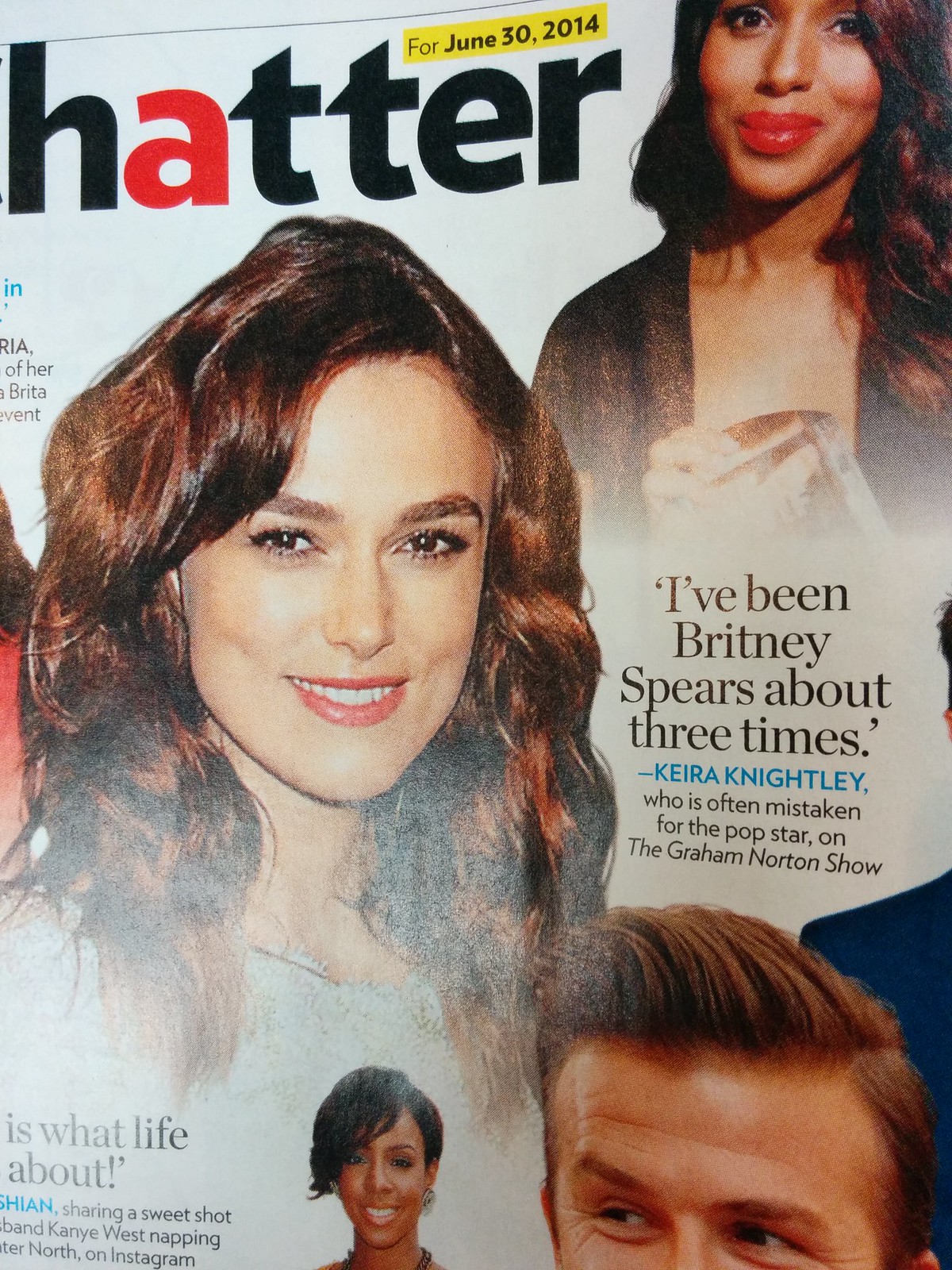The magazine cover, titled "Hatter" with the "A" in red and the remaining characters in black, features a predominantly white background. Above the "T" and "R" of "Hatter," a small yellow box announces the date, "For June 30, 2014." The main image is a large photo of a woman with long brown curly hair and white skin, smiling and looking forward at an angle—identifiable as Keira Knightley. In the top right corner, the face of another woman with dark or light brown curly hair and some text around her are partially visible. At the bottom right is the top of a man's head, hair gelled and curved to the left, most likely referring to David Beckham. Text below the image of Keira Knightley in blue recounts a quote attributed to her, often mistaken for Britney Spears on "The Graham Norton Show." A woman with short black hair, smiling and looking forward, is centered at the bottom of the cover. Additional text in the bottom left corner of the cover speculates, "Is what life about," possibly referring to a shared photo of Kanye West napping with North on Instagram.